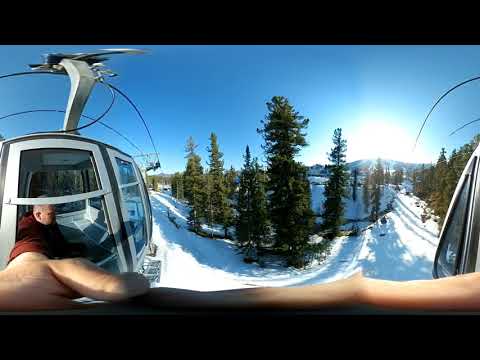The photograph, taken from within a gondola ski lift, captures a moment high above a snowy landscape. Inside the gondola, partially visible, is a man extending his arm out, possibly holding a selfie stick to take this unique, somewhat distorted, perspective. Below the gondola, a pristine ski slope or densely forested area blanketed in packed snow stretches out, with tall pine trees standing sentinel, some cleared to accommodate the gondola's path or ski trails. The bright, dazzling sun dominates the blue sky, creating a radiant halo of turquoise light around it while casting significant shadows on the snow-covered ground below. The upper and lower edges of the photograph are bordered by black bars, framing this serene, sunlit winter scene.